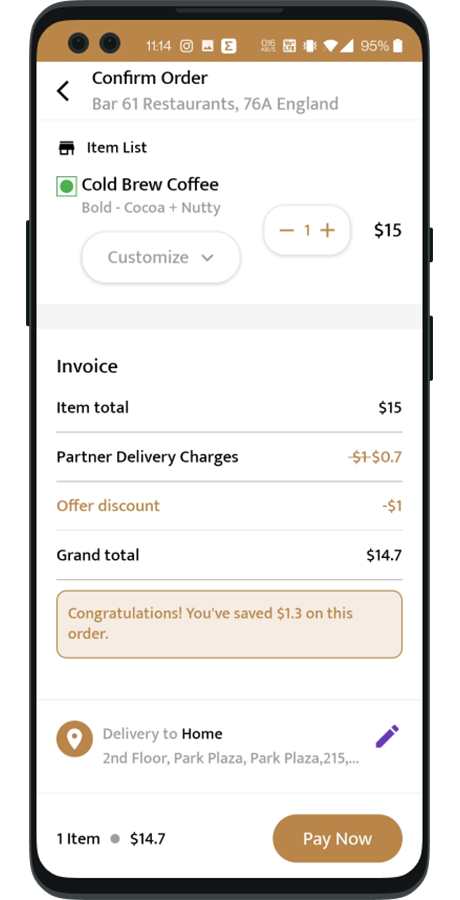**Order Confirmation Screen for Cold Brew Coffee on Mobile App**

The image depicts a mobile app screen designed for confirming an order from Bar 61 Restaurant, located at 76A England. The app prominently displays the text "Confirm Order at Bar 61 Restaurant, 76A England," indicating the order's details. The ordered item is a "Cold Brew Coffee" with a description noting it has bold cocoa and nutty flavors. The quantity selected is one, priced at $15, with a $1 discount applied. The item description and the grand total, which is $14.70, are shown below. A congratulatory message highlights that the user has saved $1.30 on the order.

The delivery information specifies the home address as "Second Floor, Park Plaza, 215." There is an option to edit the address, represented by a pencil icon adjacent to it. The order summary reiterates the total amount due as $14.70 for one item, and a prominent "Pay Now" button is displayed for finalizing the payment.

The description then digresses briefly into commentary, reflecting on the convenience of ordering a $15 coffee to be delivered to the second floor of Park Plaza, suggesting a juxtaposition between areas with such services and those where coffee places have closed due to lack of business, hinting at broader economic factors such as fast-food monopolies.